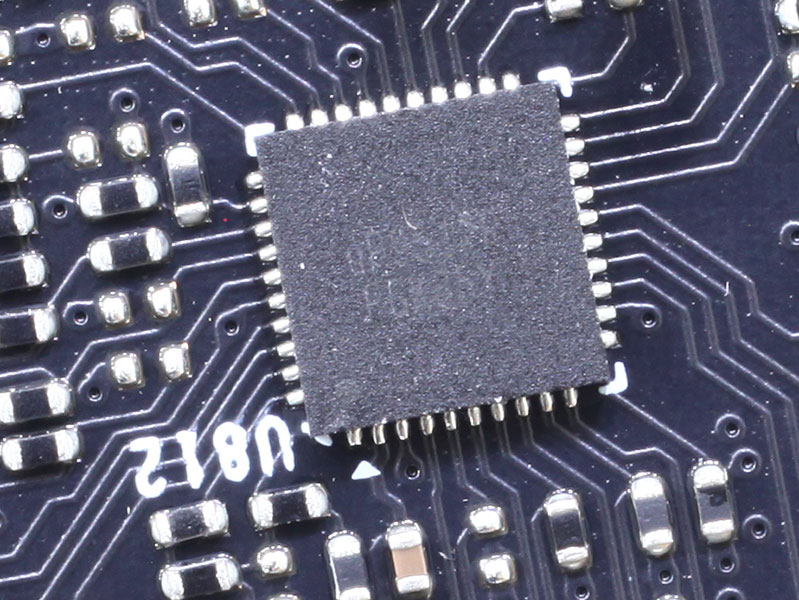This image is a detailed photograph of a dark gray circuit board, showing a prominent square microchip positioned right in the center. The chip has numerous small metallic "teeth" protruding from its edges, connecting to various points on the board through intricate silver soldered connections. Surrounding the chip are multiple components, including silver and black metal squares, pill-shaped rectangles, and other small connectors, which likely include transistors. The circuit board itself features a network of raised electrical lines that link these components, creating a complex web of connections. There is visible labeling on the board, including an upside-down inscription "U812" located in the bottom left section. The entire composition of the photograph highlights the intricate and detailed nature of the electronic circuitry.